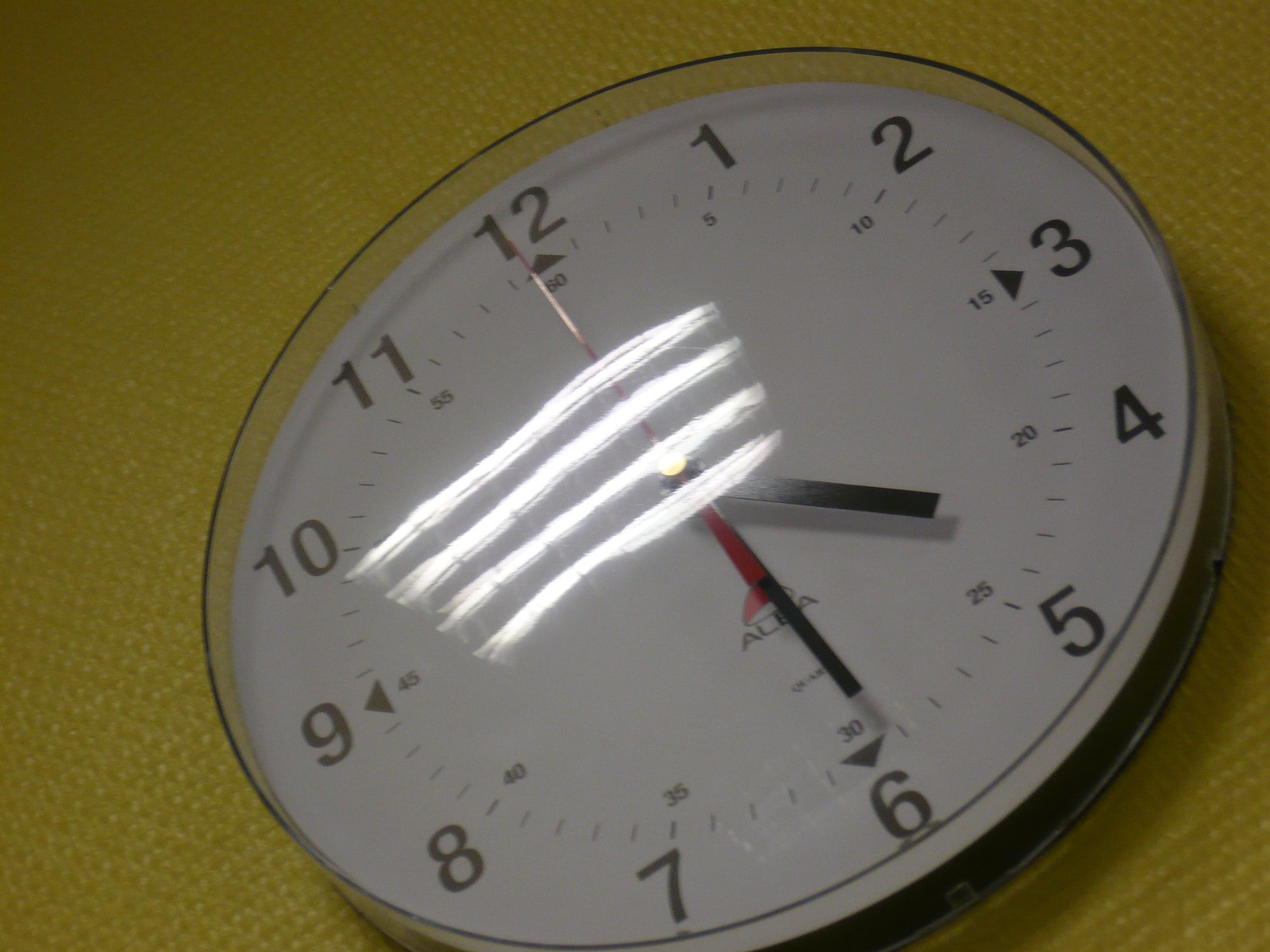The photograph depicts an institutional wall clock mounted on a pale gold, tightly woven wallpaper. The clock face, which is white with black hour and minute hands and a red second hand, is tilted so that the number 12 points slightly to the upper left. The time displayed is precisely 4:30. The clock features large black numbers from 1 to 12, with smaller numbers beneath them indicating the minutes (e.g., 5, 10, 15, etc.). Surrounding the clock face is a plastic or glass cover, reflecting four diagonal fluorescent light streaks originating from the lower left to the upper right, just right of center. The manufacturer's name, partially obscured by the clock hands, seems to start with "AC." The clock's face and numbers are clearly visible despite the reflections and slant.